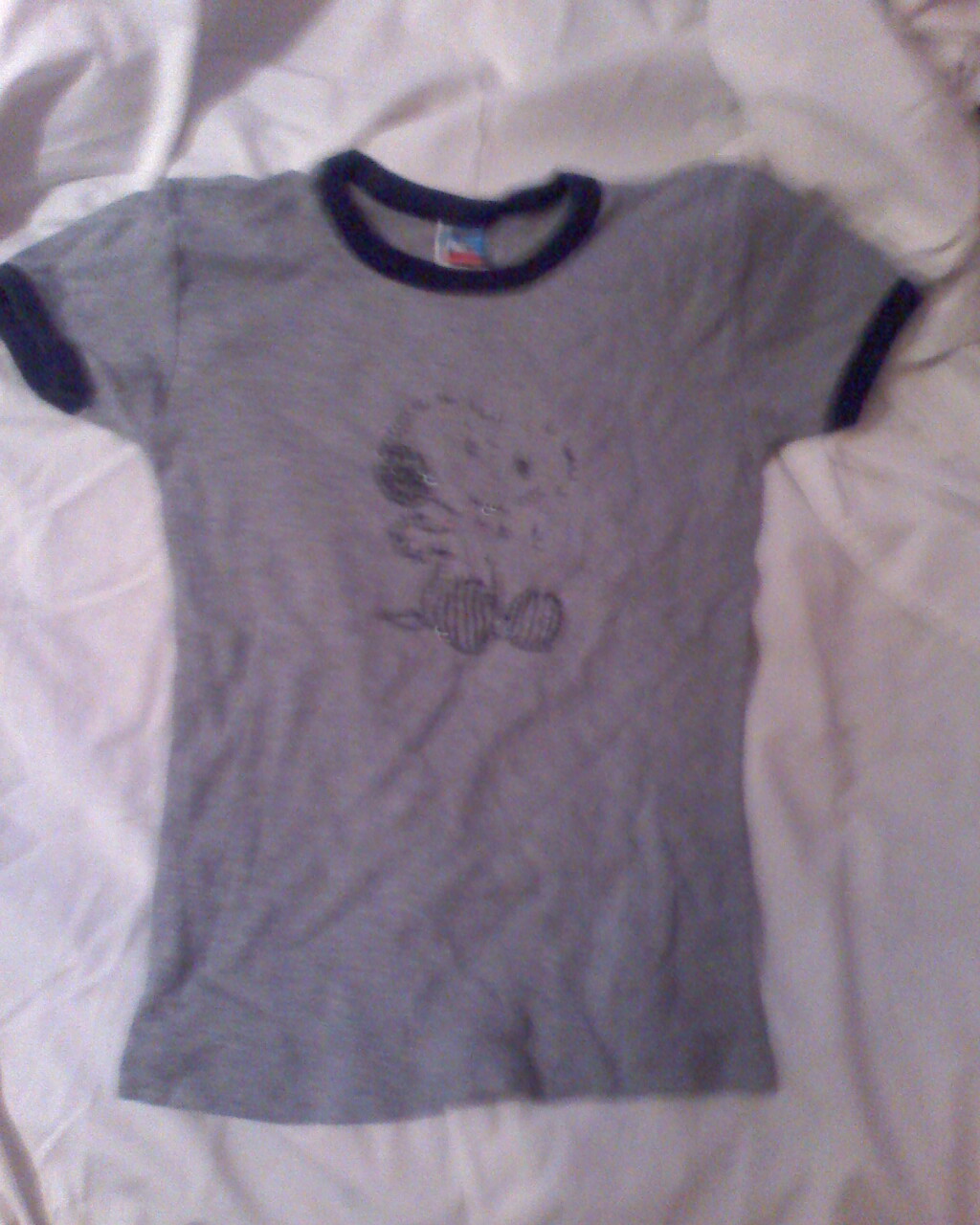This image is a very blurry photograph of a gray, short-sleeved, ringer t-shirt with blue trim around the sleeves and neckline. The centerpiece of the shirt features a smiling Snoopy sitting with his feet facing to the right and arms outstretched. His shoes display a design with intersecting lines resembling crosses. There is a red, white, and blue tag on the inside of the neck, though the script is not legible. The t-shirt appears to be placed on a wrinkled off-white or potentially pink sheet, suggesting it might be prepared for a photograph, possibly for selling online.